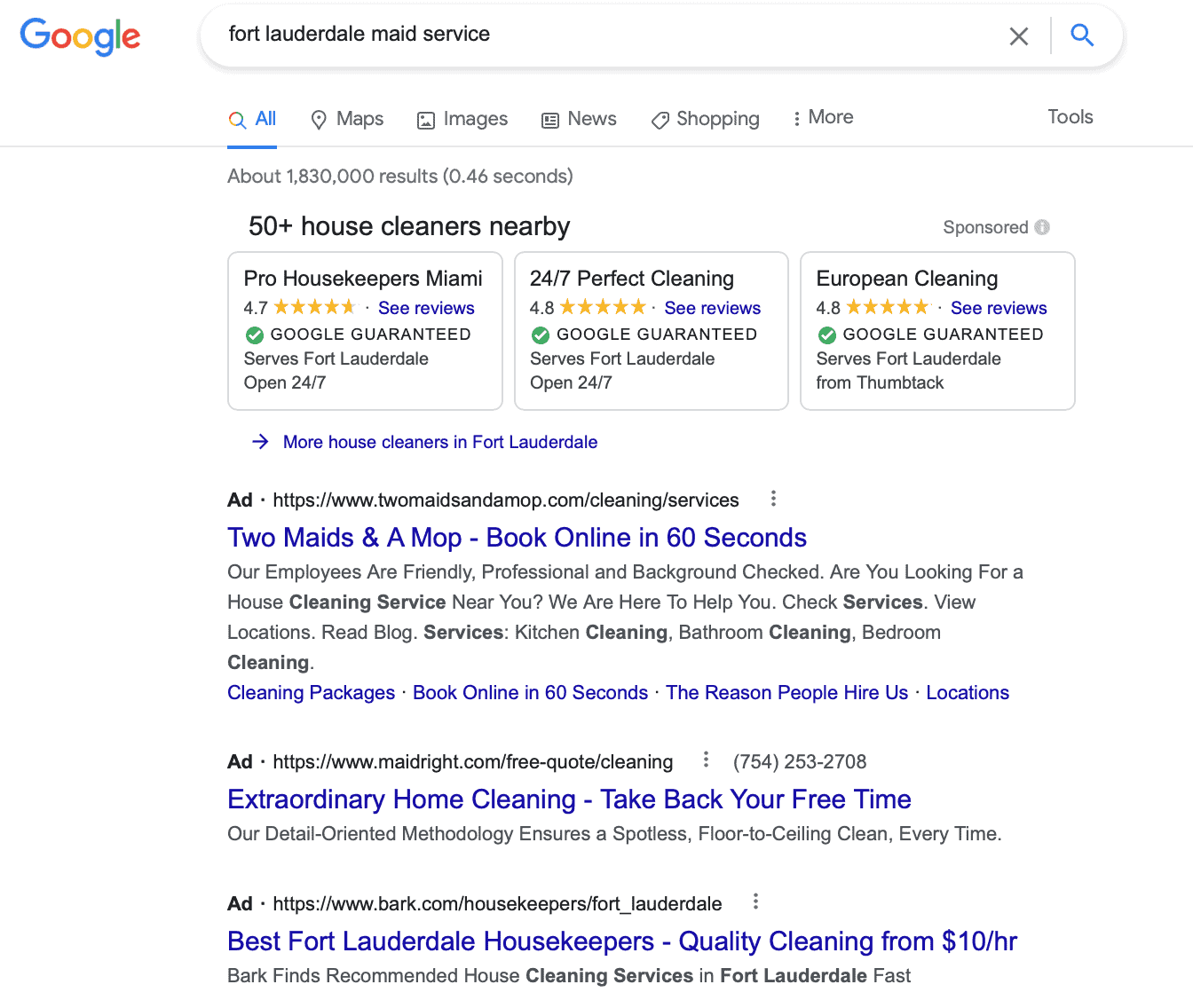The image depicts a Google search results page with the query "Fort Lauderdale maid services" displayed in the search box. The familiar Google logo, with its distinctive blue "G", red "o," yellow "o," blue "g", green "l", and red "e," appears in the top left corner. Below the search box, various categories such as "All," "Maps," "Images," "News," "Shopping," and "Tools" are listed, with the "All" category highlighted in blue while the others remain in black. The results indicate there are approximately 1 million entries, with detailed results numbering around 30,000, retrieved in 0.46 seconds.

The displayed content includes a mix of search results and sponsored ads for house cleaning services in Fort Lauderdale. Among the sponsored entries:

1. **Pro Housekeeping, Couch Keepers Miami**: Rated 4.7 stars, Google Guaranteed, and available 24/7 in Fort Lauderdale.
2. **24x7 Perfect Cleaning**: Rated 4.8 stars.
3. **European Cleaning**: Rated 4.8 stars, noted along with an option to see more house cleaners in Fort Lauderdale.

Additional advertised entries include:

- **ToolMate and a Mop Cleaning Service**: The advertisement highlights quick online booking capabilities, suggesting users can "Book online in 60 seconds."
- **Extraordinary Home Cleaning**: Promoted with the tagline "Take back your free time" and linked to the website maderight.com.
- **Best Fort Lauderdale Housekeepers**: Marketed as offering quality cleaning services starting from $10 per hour.

This comprehensive search results page efficiently lays out options for finding professional maid services in the Fort Lauderdale area, highlighting user reviews, service availability, and easy online booking opportunities.